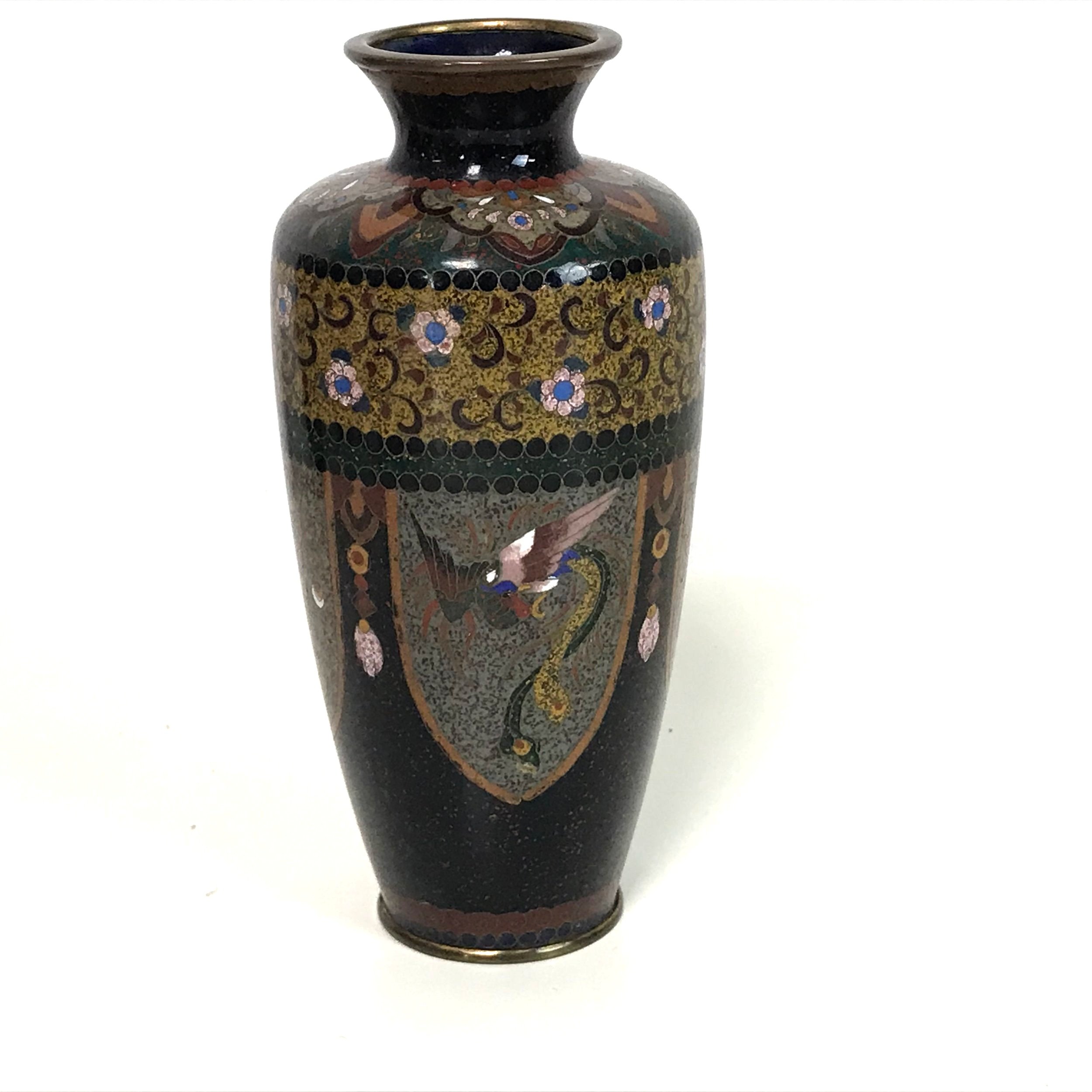The image features a tall, slender, black ceramic vessel with a glossy, polished finish. The vessel tapers in at the top, ending in a short, narrow mouth with a brown lip. It is intricately adorned with designs that include mosaic elements. On the front, there is a central depiction of a mythological creature, resembling a griffin or possibly a phoenix, situated within a grey, shield-like shape. Surrounding this are various artistic patterns, including pink flowers with dark green leaves and half-moon shapes. The palette includes dark charcoal gray, black, forest green, mustard yellow, and speckles of brown, with hints of bluish centers for the flowers and murky, musty pink-white petals. The detailed decorations extend all the way around the vessel, giving it the appearance of an ancient artifact that could be displayed in a museum. The background of the image is entirely white, fully isolating and highlighting the ornate vase.